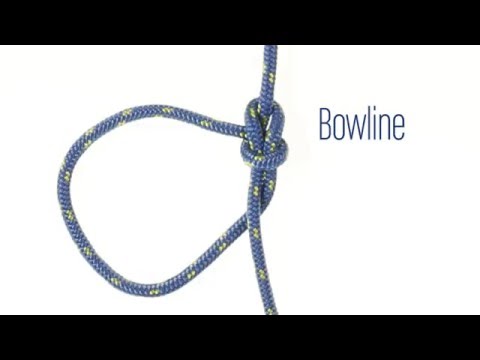The image features a single object: a piece of blue rope with evenly spaced yellow specks, arranged to demonstrate a bowline knot. The rope appears to form a loop on the left side while the main structure of the bowline is centered in the image. Notably, the knot seems loose as if it hasn't been completely tightened yet. The background is predominantly white, framed by black horizontal borders at the top and bottom, mimicking the style of an educational slide. The only text in the image is the word "bowline," displayed in a blue sans-serif font near the right-hand side, slightly below the top edge. The overall composition and style suggest that this image is intended for instructional purposes, likely to teach viewers how to tie a bowline knot.